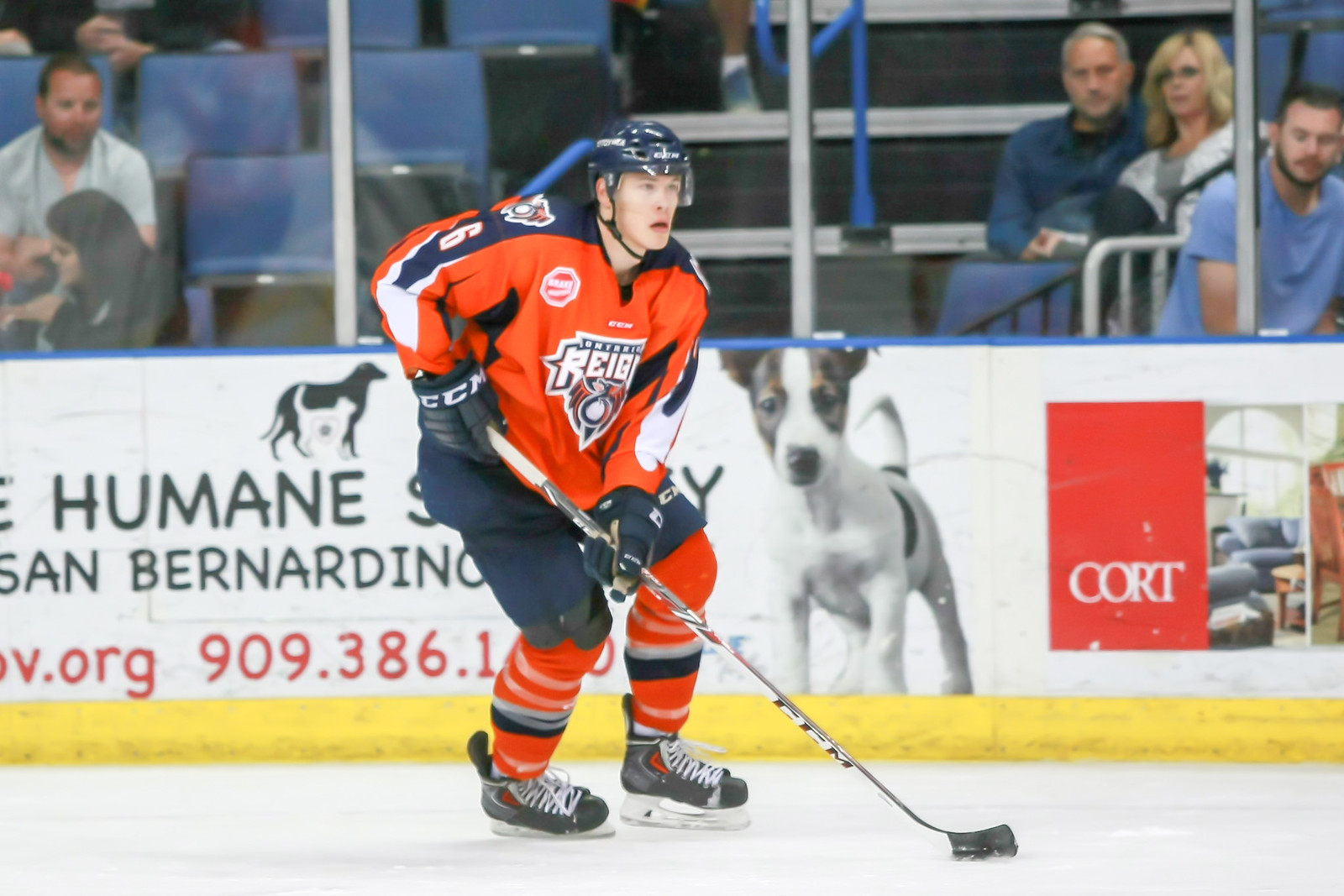The photograph captures an action-packed moment from a hockey game, likely featuring a team from the Ontario Reign, judging by the jersey design. The player at the center of the frame is skating forward, firmly gripping their hockey stick. The jersey sports a striking combination of orange and black colors. In the background, the boards are adorned with various advertisements, including a prominent one for the San Bernardino Humane Society and another for a furniture company named "Court" to the right. The stands rise just above the boards, showing about three rows of spectators. A few fans are visible on the left side of the stands, while three more can be seen on the right, adding to the lively atmosphere of the game.